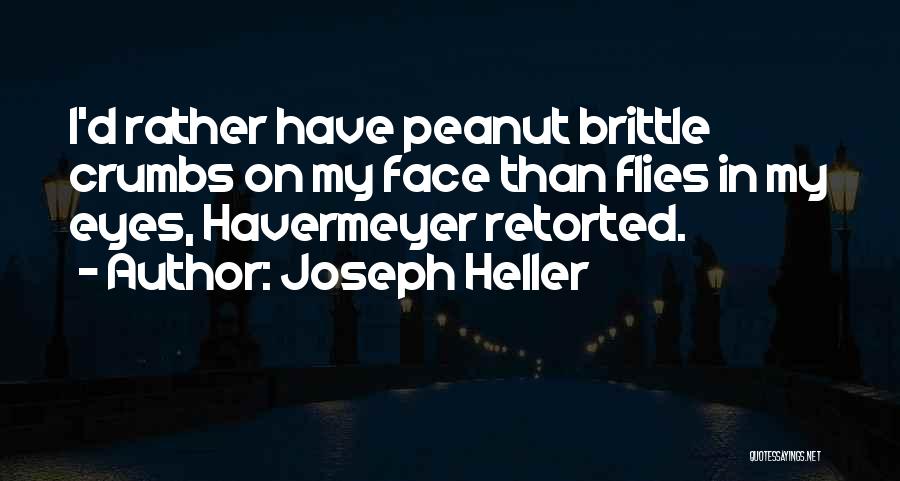The image features a very dark background, perhaps a highway or a body of water, bordered by thin, tall street lamps with black columns and warm lanterns at the top. These lamps line both sides of what seems to be a road, converging towards the center of the image, forming an almost V-like shape from the bottom center to the vanishing point in the distance. The dark navy sky enhances the shadowy atmosphere, while the lit street lamps cast a warm yellow glow on the surroundings. In the middle-left portion of the image, slightly above the center, there is a white text quote left-aligned across four lines: "I'd rather have peanut brittle crumbs on my face than flies in my eyes, Havermeyer retorted." Below this quote, a line reads "- author: Joseph Heller." In the lower right corner, in very small white font, the source "quotes.sains.net" is noted, being barely one-fifth the size of the main text.